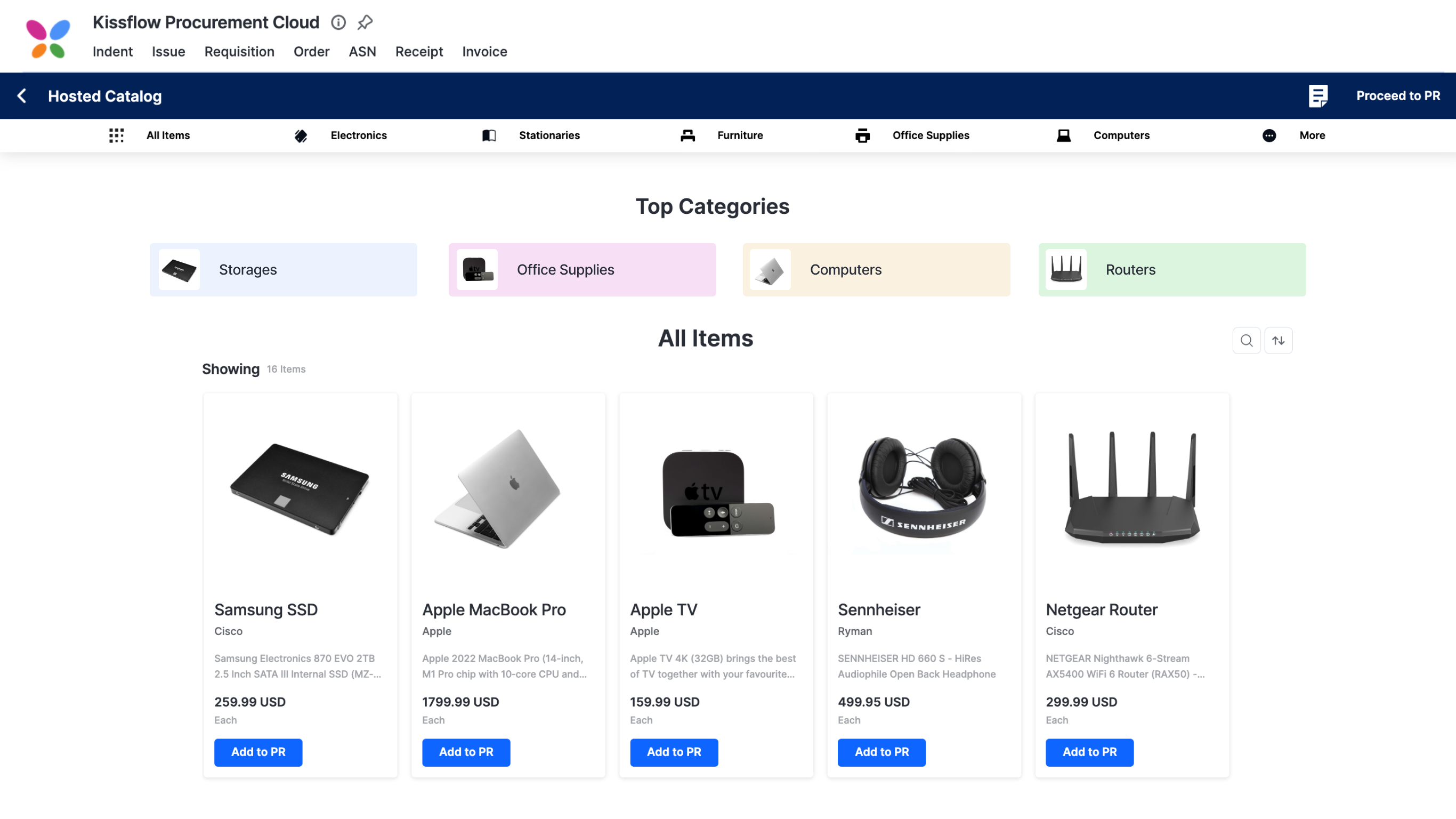This image showcases a webpage from the KISS Flow Procurement Cloud, an online platform for purchasing various items. The top of the webpage features a navigation menu with options labeled: Indent, Issue, Requisition, Order, ASN, Receipt, and Invoice. A secondary navigation bar includes links to different sections: Hosted Catalog and Proceed to PR.

Below these navigation bars, the main interface is divided into several clickable categories for streamlined shopping, including All Items, Electronics, Stationery, Furniture, Office Supplies, and Computers. Additional categories can be accessed via a "More" button.

The bottom section of the webpage displays "Top Categories," segmented by color-coded rectangles: Storage (blue), Office Supplies (lavender), Computers (tan), and Routers (green). Displayed beneath this section are images and names of five featured products: an Apple MacBook Pro, a Samsung SSD card, an Apple TV, a Sennheiser headset, and a Netgear router.